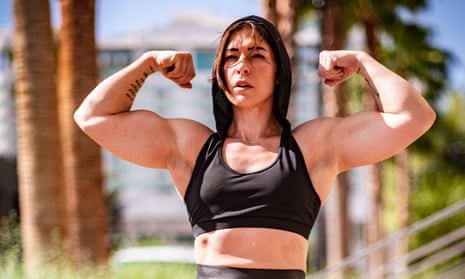In this photograph, a very muscular woman poses confidently, showcasing her impressive bicep muscles as she holds both arms up with clenched fists. She is wearing a black sports bra and tight, black waistband shorts or pants. Her skin is quite pale, indicating she might be Asian or Caucasian. She has long, straight, dark brown shoulder-length hair and a serious expression on her face. Notably, her right forearm features a tattoo comprised of six or seven black lines. 

The background includes a slightly blurry building, green grass, and several palm trees against a blue sky, signaling a pleasant day. White diagonal lines appear in the bottom right corner of the image. The photograph is cropped to show her from the top of her head to her waist. Overall, she looks incredibly strong, with a well-defined, athletic physique that could make her competitive in a boxing or bodybuilding competition.